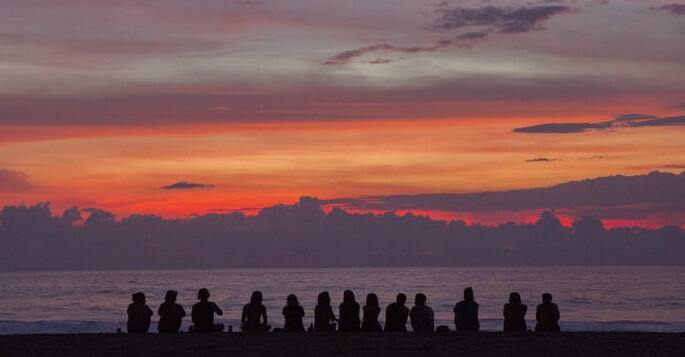This photograph captures an enchanting outdoor scene of people enjoying a sunset at the beach. In the foreground, the silhouettes of about 10 to 15 individuals are seen lined up, sitting on the dark sand. Their backs are towards the viewer, making them appear as shadowy outlines. Beyond the seated figures lies a flowing body of water with a dark blue hue, while the far edge of the water features a landscape or hill, now dimmed to a purple-gray shade by the setting sun and dusk.

The sky is a breathtaking gradient of colors, with dark gray clouds near the horizon. As the eye moves upward, the sky transitions through deep reds, vibrant oranges, and yellows, ultimately fading into light blue at the top. Wispy, misty clouds intermingle with these hues, adding to the overall ethereal quality of the scene. The unique, colorful sky not only enhances the silhouettes of the people but also adds a magical ambiance to this moment captured in time.